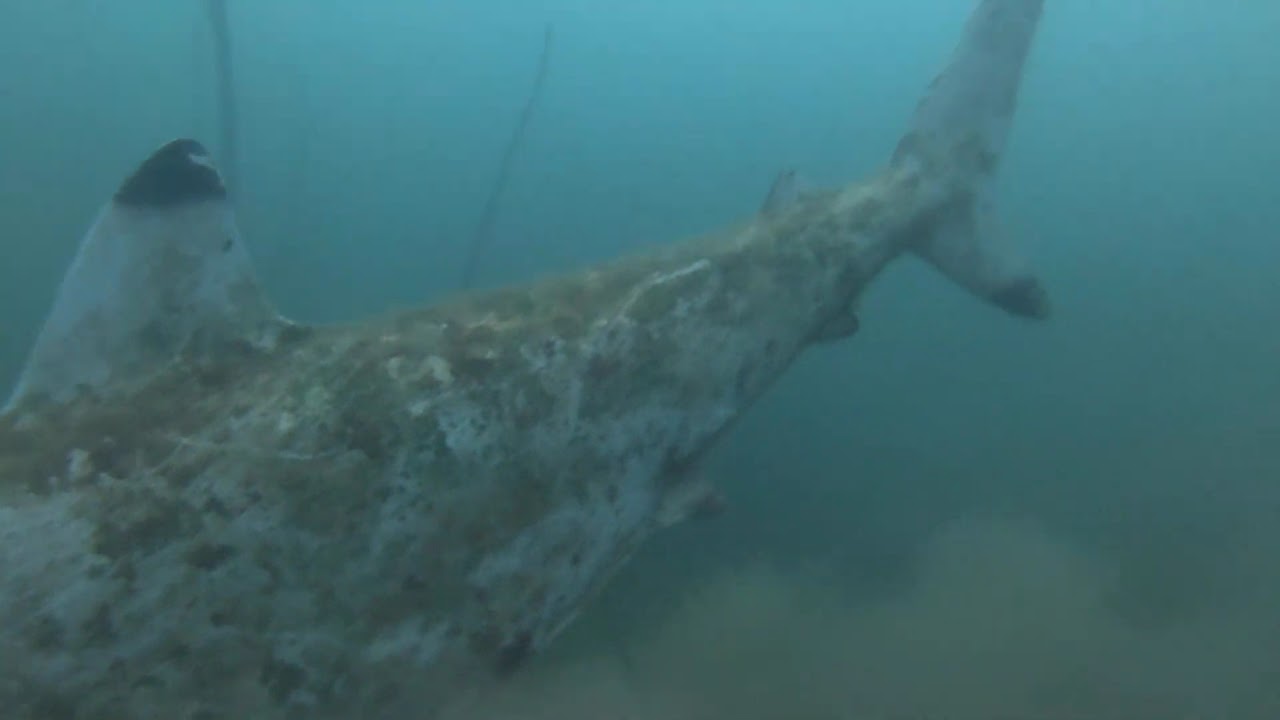This underwater image is taken quite a ways below the surface and appears distorted, lending a hazy, light blue tint to the overall scene. The main focus of the image is a large fish, likely a shark or whale, seen from the tail end and extending up to just before the dorsal fin. The creature has a moldy appearance with a combination of white, brownish, black, and greenish colors, possibly suggesting a diseased state or natural patterning. The fish's tail and dorsal fin are clearly visible, pointing to its sizable presence in the frame. Surrounding the fish, the water appears foggy with sand or debris kicked up at the bottom, and two thin, dark streaks are noticeable in the background. Additionally, there are a few stalks of kelp growing up from the ocean floor, hinting that this scene captures a moment within a kelp forest.